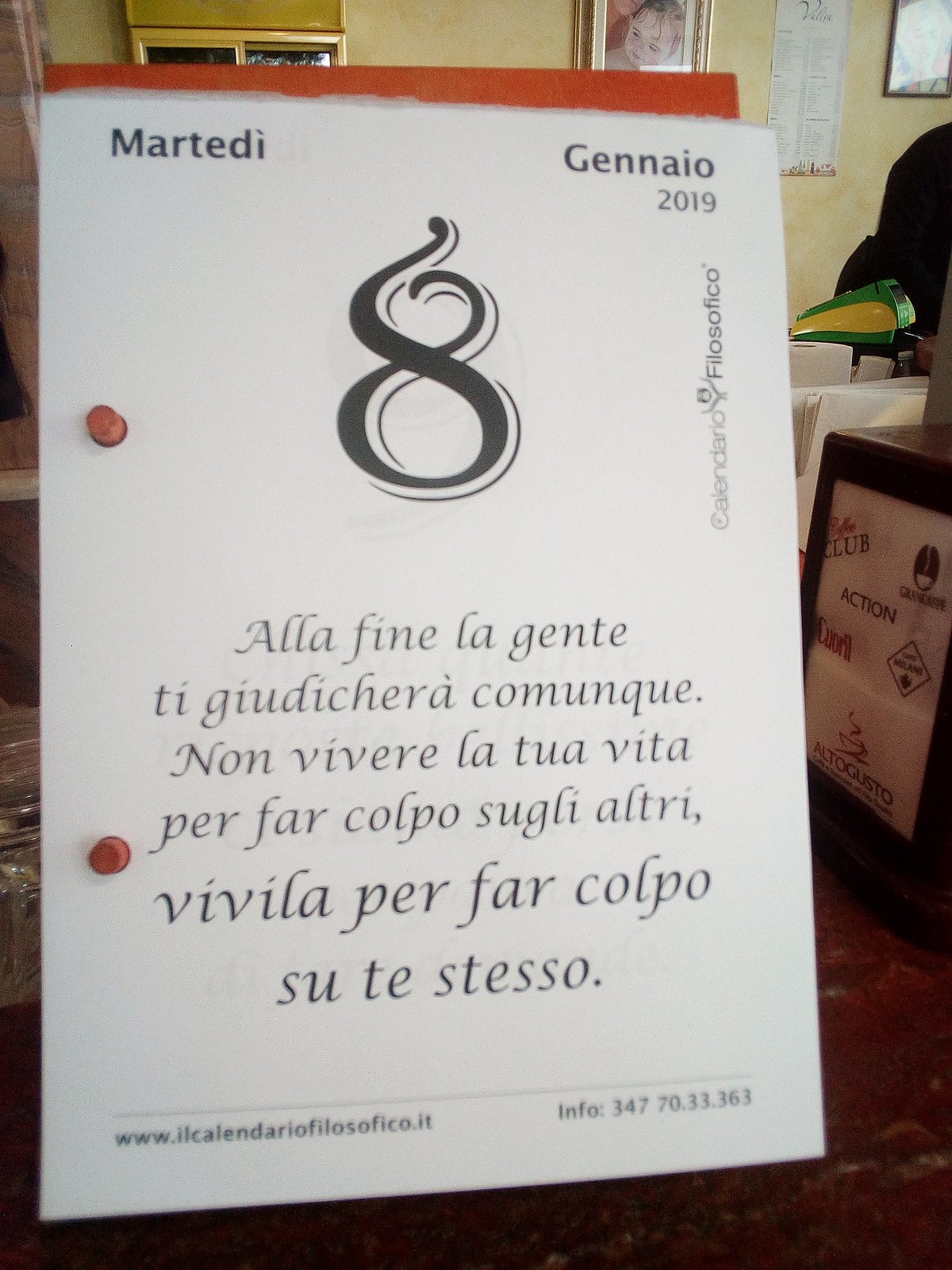This is a vertical rectangular photograph of a tear-off page from an Italian calendar of philosophy, specifically dated January 8, 2019. The page is slightly diagonal, with the top leaning to the left and the bottom to the right, bound by red posts at the side and a red top binding. In the upper left corner, it reads "Martedì," and on the right, "Gennaio 2019." Dominating the center of the page is a large, elaborate number "8" in black and white. Below the number is an Italian quote: "Alla fine la gente ti giudicherà comunque, non vivere la tua vita per far colpo sugli altri, vivila per far colpo su te stesso," which translates to "In the end, people will judge you anyway, so don't live your life to make an impression on other people, live it to make an impression on yourself." At the bottom, a line separates this saying from the website "www.ilcalendariofilosofico.it" and additional information, including a mobile number, "347-70-33-363." The background reveals part of an interior space, possibly a house or office, with pictures on the wall contributing to the homely ambiance.